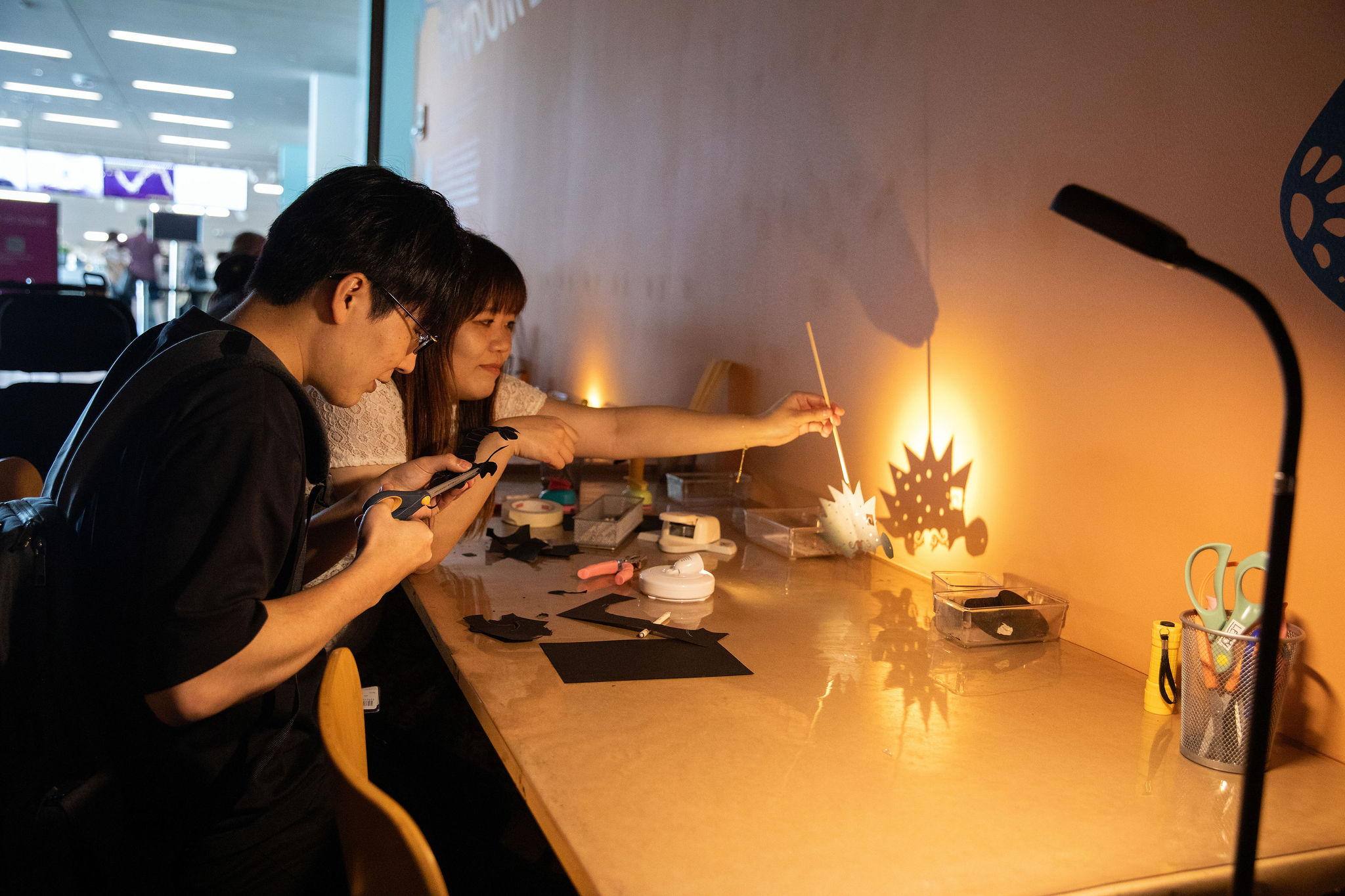In this landscape-oriented photograph, two people of Asian descent are engaged in a crafting activity, likely within an office or animation studio setting. Both are seated at a long desk cluttered with crafting supplies and small acrylic boxes. The man, dressed in black, is on the right side and is carefully cutting out shapes from a black piece of paper with scissors. Sitting next to him, the woman, wearing a white shirt and with long dark hair, is holding a skewer stick to which she has attached a cardboard cutout that resembles a vehicle with ridged tops and holes, evocative of an animal or cartoonish creature. They are projecting a light source onto the cutout to cast a shadow on the wall, experimenting with the shadow as part of the creative process. Overhead lights illuminate the spacious office, where other people can be seen working in the background.